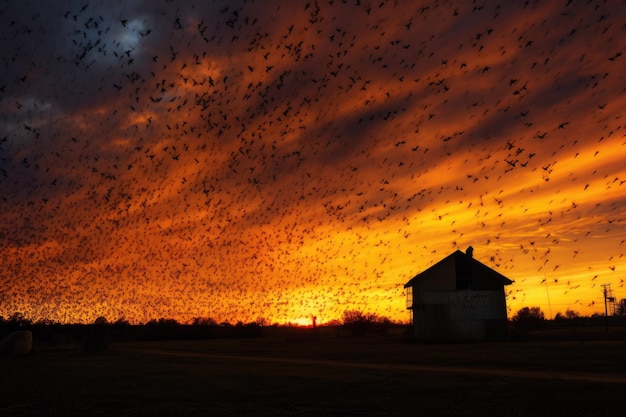This captivating image captures the dramatic beauty of an outdoor sunset scene. The sky is a mesmerizing gradient, transitioning from deep purples and dark blues in the top left corner to vibrant yellows and fiery oranges across the rest of the sky, culminating in a burnt orange at the horizon line. Silhouetted against this brilliant backdrop is a sprawling landscape that features the shadowy outlines of a forest, a small house or shack situated more to the right, and what appears to be a road at the bottom. Adding to the ethereal atmosphere, a thick swarm of black birds fills the sky—tiny pinpricks that create an almost apocalyptic ambiance. These birds, flying in a unified direction, give the scene a hauntingly dynamic element, especially as they move beneath patches of darker clouds that speckle the sky. The overall effect is a stunning, albeit unsettling, juxtaposition of natural beauty and eerie motion.